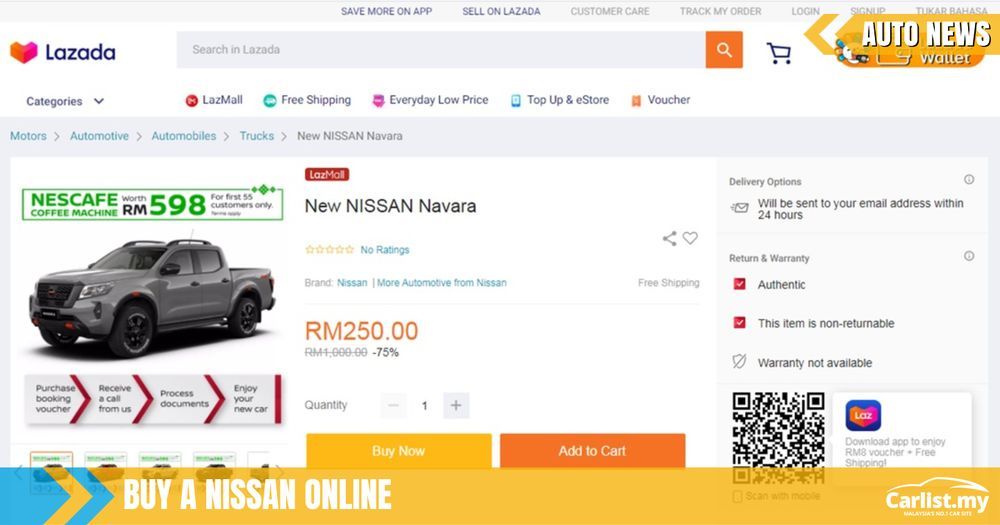Screenshot of a car shopping webpage on Lazada.

The Lazada logo, resembling an "L" laid on its side with a 3D cube effect with a cutout at the back, gives the appearance of a "V". The logo transitions from orange on the left to pink on the right. Next to the logo is a search bar with an orange search button on the right.

In the upper right-hand corner, there are sections for "Auto News" and "Wallet", indicated with prominent arrows and text. The website's navigation menu includes links to "Save More on Apps", "Lazada", "Customer Care", "Track My Order", "Log In", "Sign Up", and "Tukar Bahasa" (which may translate to "Change Language" or be a username).

Below this navigation bar is a horizontal menu featuring options like "Categories", "LazMall", "Free Shipping", "Everyday Low Price", "Top Up & eStore", and "Voucher", each accompanied by small icons.

Further down, the page presents automotive search results, specifically highlighting a new Nissan Navara truck. The truck is displayed in a three-quarter view facing left. The vehicle is a sleek grey pickup with four doors and a roof rack. 

A pop-up advertisement for a Nescafe coffee machine is visible, partially obstructing the view of the Nissan Navara.

The product listing reads "New Nissan Navara" with no customer ratings. The price is prominently displayed as RM250, down from RM1000, reflecting a 75% discount. Options to share and like the listing are provided.

On the far right, delivery options state that the item will be emailed within 24 hours. Next to it, two red-checkmarked boxes confirm that the item is under return warranty but is non-returnable.

Below the truck image, an info graphic outlines the purchasing steps: "Purchase", "Booking", "Voucher", "Receive a Call", "Process Documents", and "Join Your New Car".

At the bottom of the page, there's a banner with the text "Buy a Nissan Online", highlighted by a full yellow underline. The banner features two center-aligned buttons; a yellow "Buy Now" button on the left, and an orange "Add to Cart" button on the right.